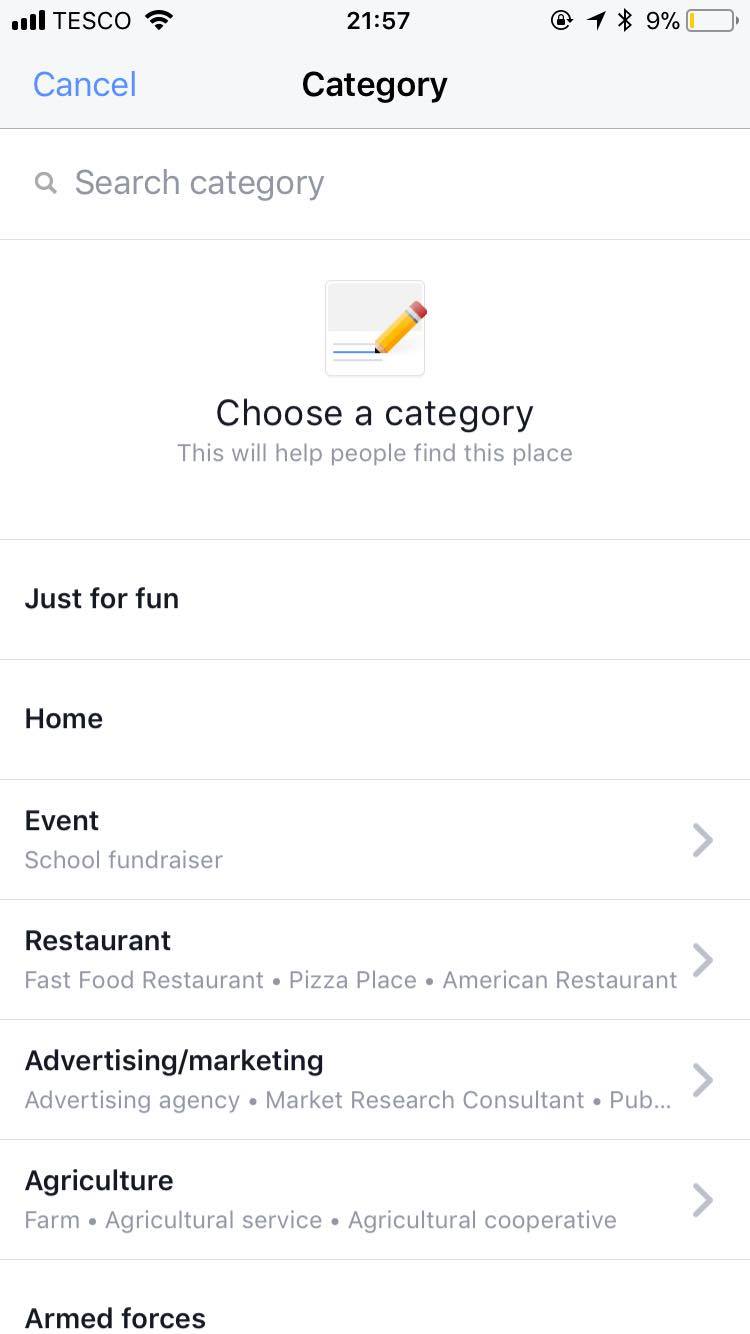The image displays a cell phone screen predominantly filled with text on a white background. The top right corner of the screen features an icon of an almost empty battery indicating 9% battery life. In the top left corner, icons for wireless and cellular connections are visible, accompanied by the text "Tesco." Beneath these icons, "Cancel" is written in blue text, aligned next to the black text "Category" in the center of the screen. 

Below this section, there is a search bar labeled "search category." Further down, there's a small square image depicting a piece of paper with a pencil writing on it, accompanied by the larger text "Choose a category," and smaller text, "This will help people find this place."

Following this, a list of categories is presented in black or gray text:
- "Just for fun"
- "Home"
- "Event" 
  - "School fundraiser" (with a right-pointing arrow)
- "Restaurant" 
  - "Fast food restaurant"
  - "Pizza place"
  - "American restaurant" (with a right-pointing arrow)
- "Advertising/Marketing" 
  - "Advertising agency"
  - "Market research consultation" (with a right-pointing arrow)
- "Agriculture" 
  - "Farm"
  - "Agricultural service"
  - "Agricultural cooperative" (with a right-pointing arrow)
- "Armed forces"

Overall, this image shows a text-heavy interface designed for selecting a category, complete with navigation aids such as search bars and right-pointing arrows for subcategories.